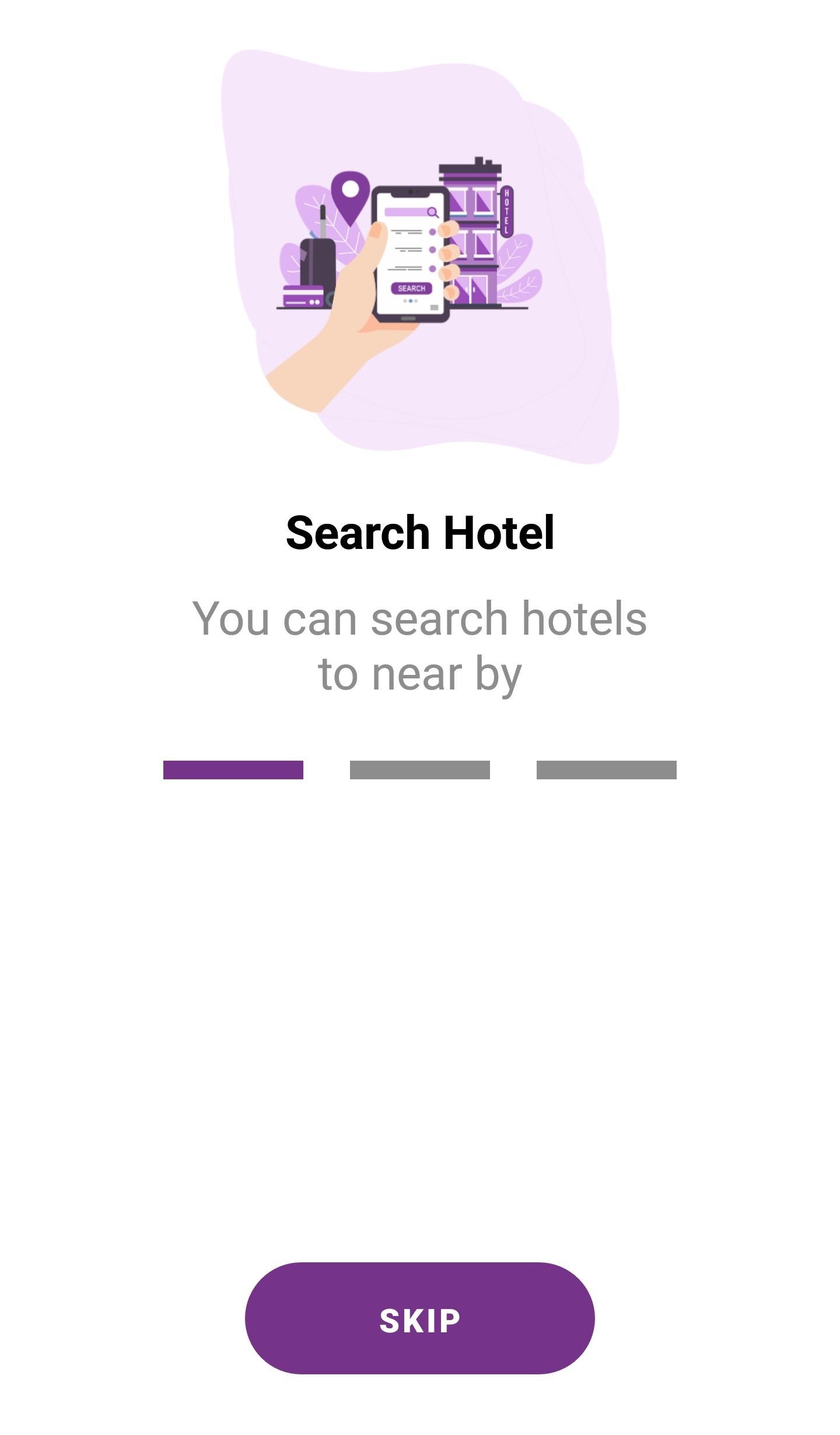The image features a white background with a light purple shading overlay at the top, depicting an animated wrist and hand holding a cell phone. At the top of the image, there are several purple icons, including a prominent location pin and a building, all maintaining a cohesive animated style. Directly beneath these icons is the text "Search hotel" in black. Below this, in gray text, it reads, "You can search hotels nearby." Further down, there are three horizontal lines: the first one is purple, while the middle and bottom lines are gray. At the bottom of the image, there is a purple section with the word "Skip" centered in white text. The entire image is encased within the white background, ensuring the elements stand out clearly.